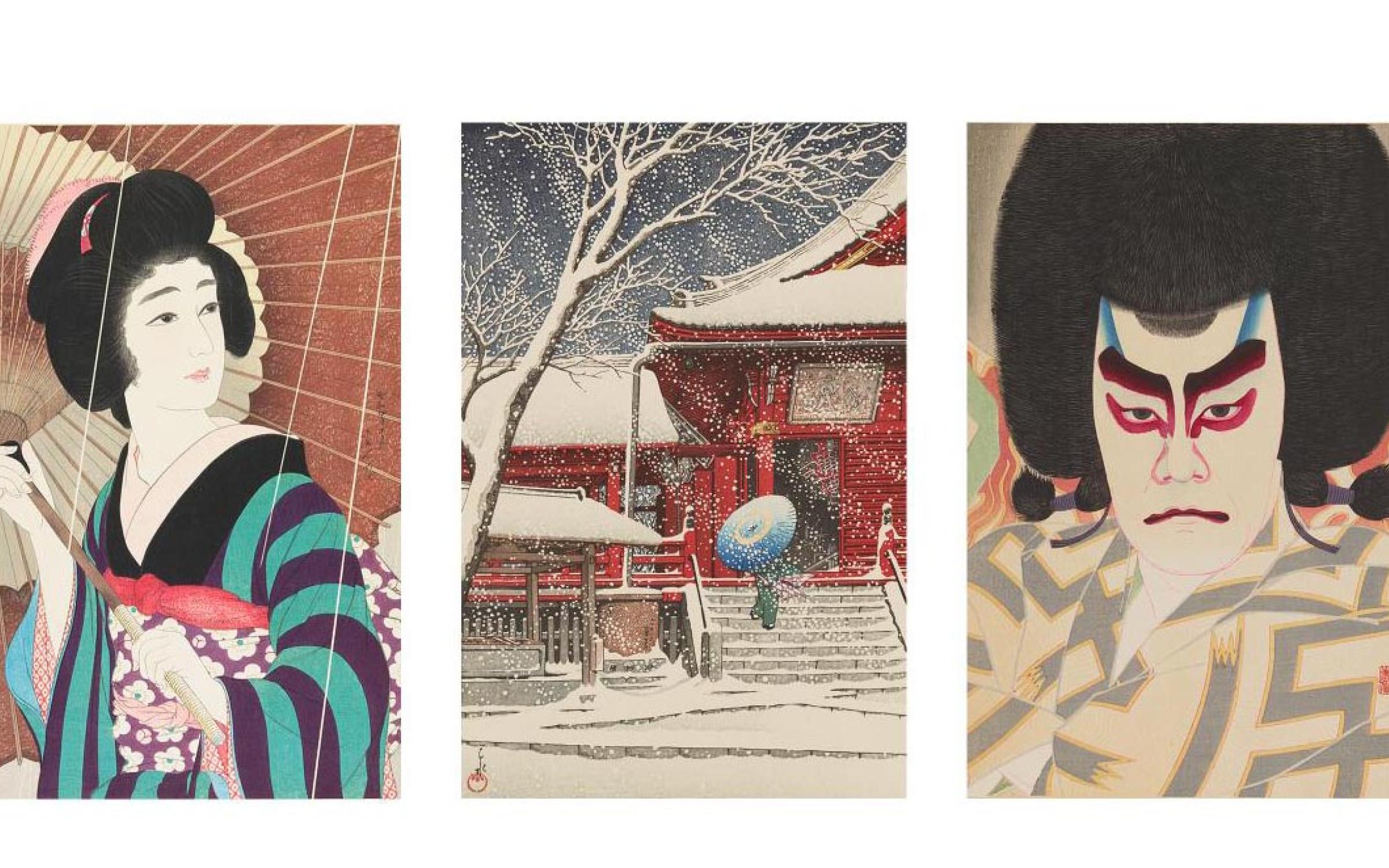This is a detailed, three-part triptych painting in a vintage Japanese artistic style. The left panel features a pale-skinned geisha dressed in a green, purple, and black floral-patterned kimono. She stands in front of a salmon-colored wall, looking towards the right, holding a fan. The middle panel depicts a red Japanese-style house during winter. Snow blankets the ground, roofs, and a bare tree reaching towards the house. A person in a green outfit and holding a blue umbrella descends the eight or ten steps leading to the open door. The right panel portrays a man, possibly a samurai, with long black hair and red makeup accentuating his eyes and eyebrows. He wears a gray-patterned kimono and has a scowling expression, possibly implying he is looking at the geisha entering the house. This triptych collectively evokes a narrative through its harmonious yet individually distinctive scenes.